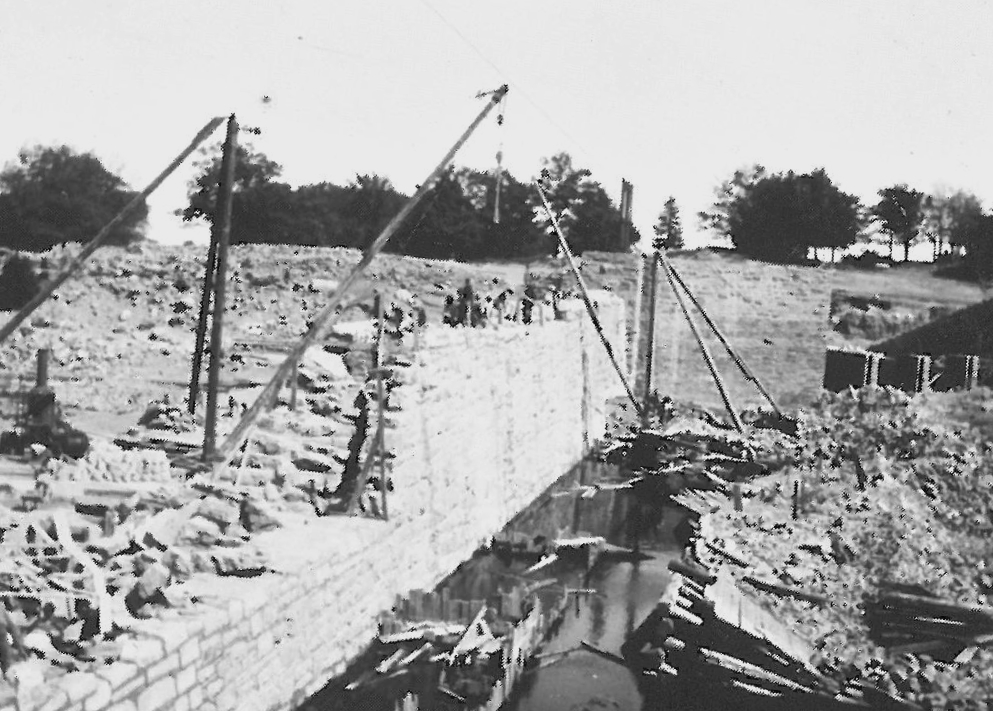This black-and-white vintage photograph, captured in landscape orientation, portrays a construction site amidst a backdrop of a clear, gray sky devoid of clouds. Trees thick with leaves line the horizon, creating a natural border around the scene. The focus is on a chaotic but structured area filled with various industrial materials and remnants. On the left side of the image, there's a substantial amount of rubble and dirt, alongside three poles arranged in a triangular, teepee-like formation. This section also features cranes and dangling pulleys, suggesting ongoing construction activities.

Towards the center, the interior of a partially completed room or space is evident, cluttered with dirt, wooden pallets, and planks. An overpass made of brick transitions from the background to the foreground, where a half-completed and jagged brick wall connects, its height diminishing towards the left. Leaning poles and additional construction materials add to the sense of turbulent activity. On the right side of the image, a bank of dirt abuts an area resembling an old log chute site with visible water flow. Above this area, another straight wall runs parallel to the horizon, enhancing the structural depth of the scene. The photograph superbly encapsulates the realism and detail of vintage black-and-white photography, offering a vivid glimpse into the industrial environment of the past.